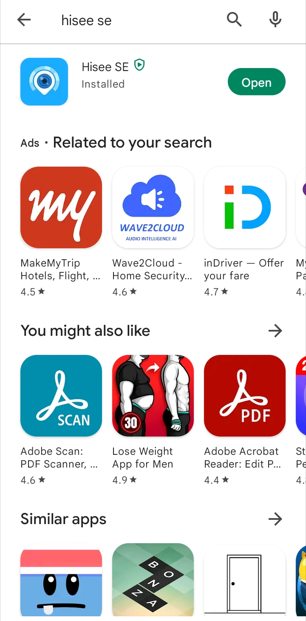The image is a cropped screenshot of the App Store as viewed on a cell phone. The search bar at the top left contains the text "hisee se," though it appears to have been meant to be "hicc." Below the search bar, an app icon is visible on the left, with the app name "hicse" to its right, followed by the word "installed." On the far right side of this app listing, there is a green "Open" button. 

Directly beneath this, the word "Ads" appears in small black letters on the left side, and "Related to your search" is prominently displayed in larger black letters to the right. Under this section, there is a horizontally scrollable row featuring three app icons for additional apps related to the search.

Continuing further down the screenshot, the text "You might like" introduces another set of thumbnails or icons for recommended apps. At the very bottom of the image, there is a "Similar apps" section with a white circle displaying an arrow pointing to the right; clicking this would expand the category to reveal more similar apps.